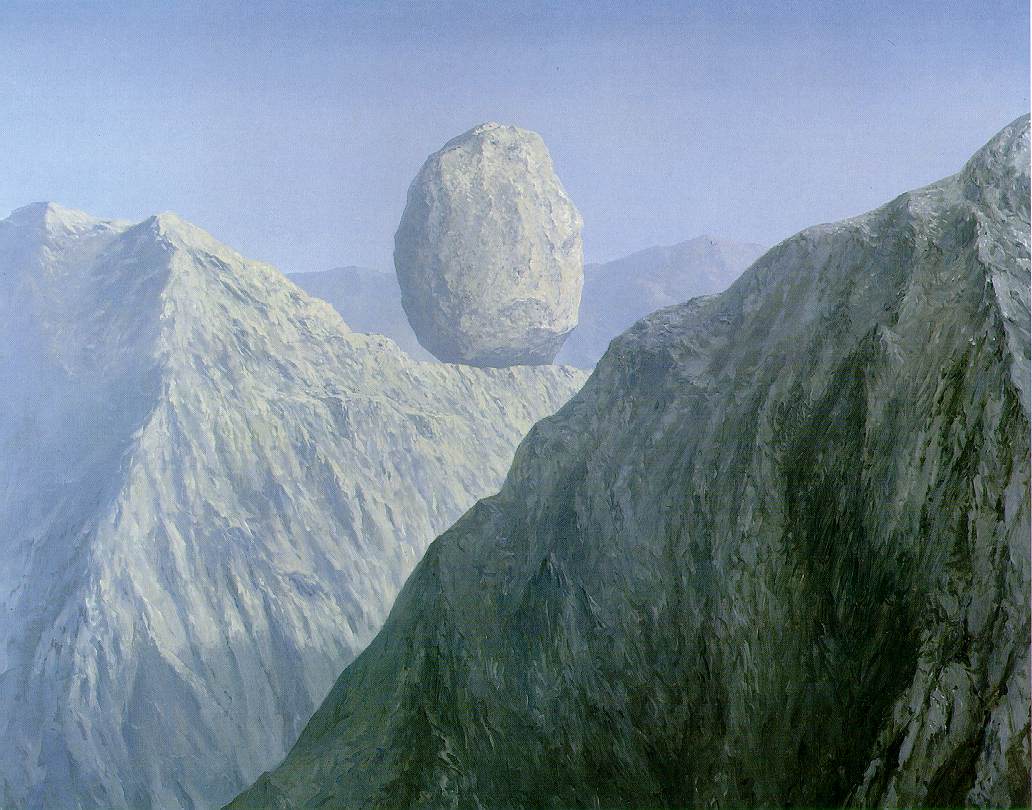The image features a surreal, possibly computer-generated scene dominated by a range of mountains under a hazy blue sky. The foreground on the right side showcases a very dark mountain, extending diagonally from the top right to the bottom left of the image. To its left, there's a lighter-colored mountain, suggesting it might be snow-covered, which intersects the dark mountain and extends upwards and off the page at the upper left corner. A prominent feature is an egg-shaped boulder perched precariously near the center, appearing almost as if it's floating. In the background, additional faint, distant mountain peaks add depth to the landscape, creating layers of mountains that occupy around 70-80% of the image. The overall scene is both serene and enigmatic, with the central boulder adding a sense of imbalance and intrigue.